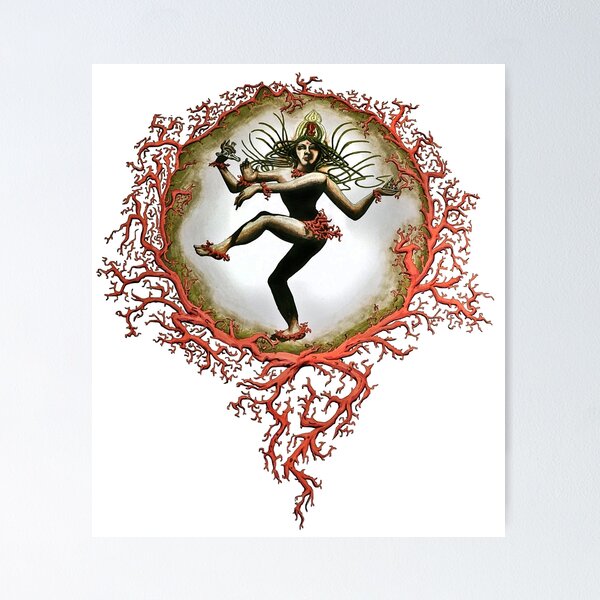This image portrays an intricate painting set against a plain white background, positioned on a light gray surface without a frame. The central feature is an orb, encircled and cradled by a dramatic, pink salmon-colored bramble or thornbush. This circular bramble extends downwards, forming a tail or handle that anchors the orb to the background. The orb itself transitions from a light center to darker shades of green towards its edges, blending with the surrounding thick brambles.

Inside the orb resides a fascinating figure, possibly a dancing god or goddess, depicted with a humanoid form but possessing four arms and two legs, one of which is raised gracefully. This figure is adorned with elaborate and wiry elements reminiscent of a headdress and is entwined with pieces of the surrounding salmon-colored thornbush. The entity's body is detailed with a black outfit that includes twig-like or stick-like accessories around its waist, feet, and arms, creating a loincloth-like appearance. Long, wispy, vine-like hair or elements extend from the head, adding to the mystical aura. 

Overall, the painting is a unique and captivating piece, blending elements of nature and deity-like figures in a dance of motion and elaborate decoration.